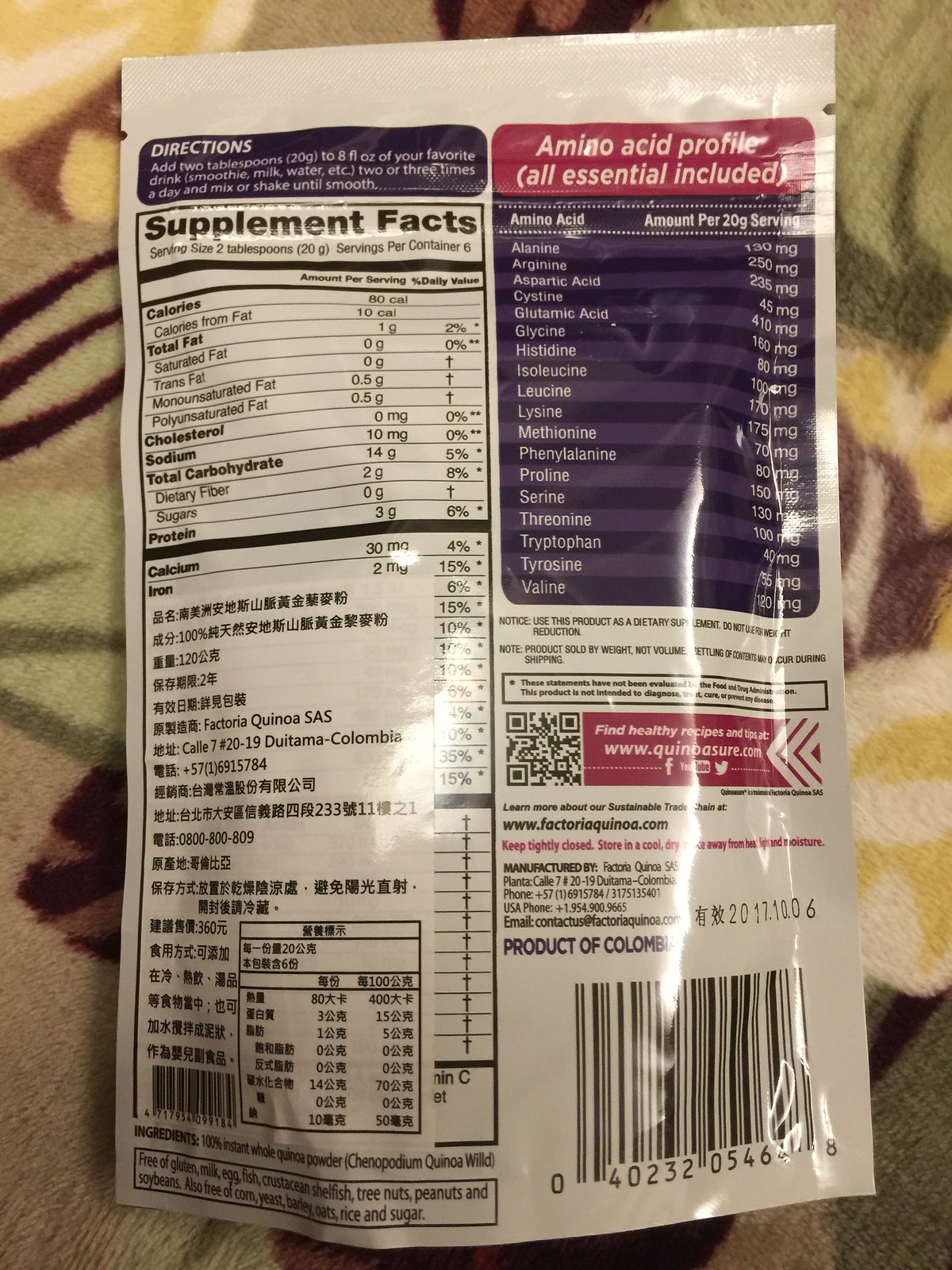The image is a photograph capturing the back side of a white food package, which appears to be some type of dietary supplement. The package features red and blue labeling. At the top of the package, there are directions instructing users to "add two tablespoons to your favorite drink, two or three times a day," and to "mix or shake until smooth." Below these instructions, there is an amino acid profile and a nutrition label, confirming that the product is indeed a supplement, as indicated by the "Supplement Facts" section. Additionally, the packaging notes that the product is manufactured by a company named Factoria Quinoa, suggesting that the supplement might be quinoa-based. The front of the package is not visible, leaving the specific type of supplement unknown.